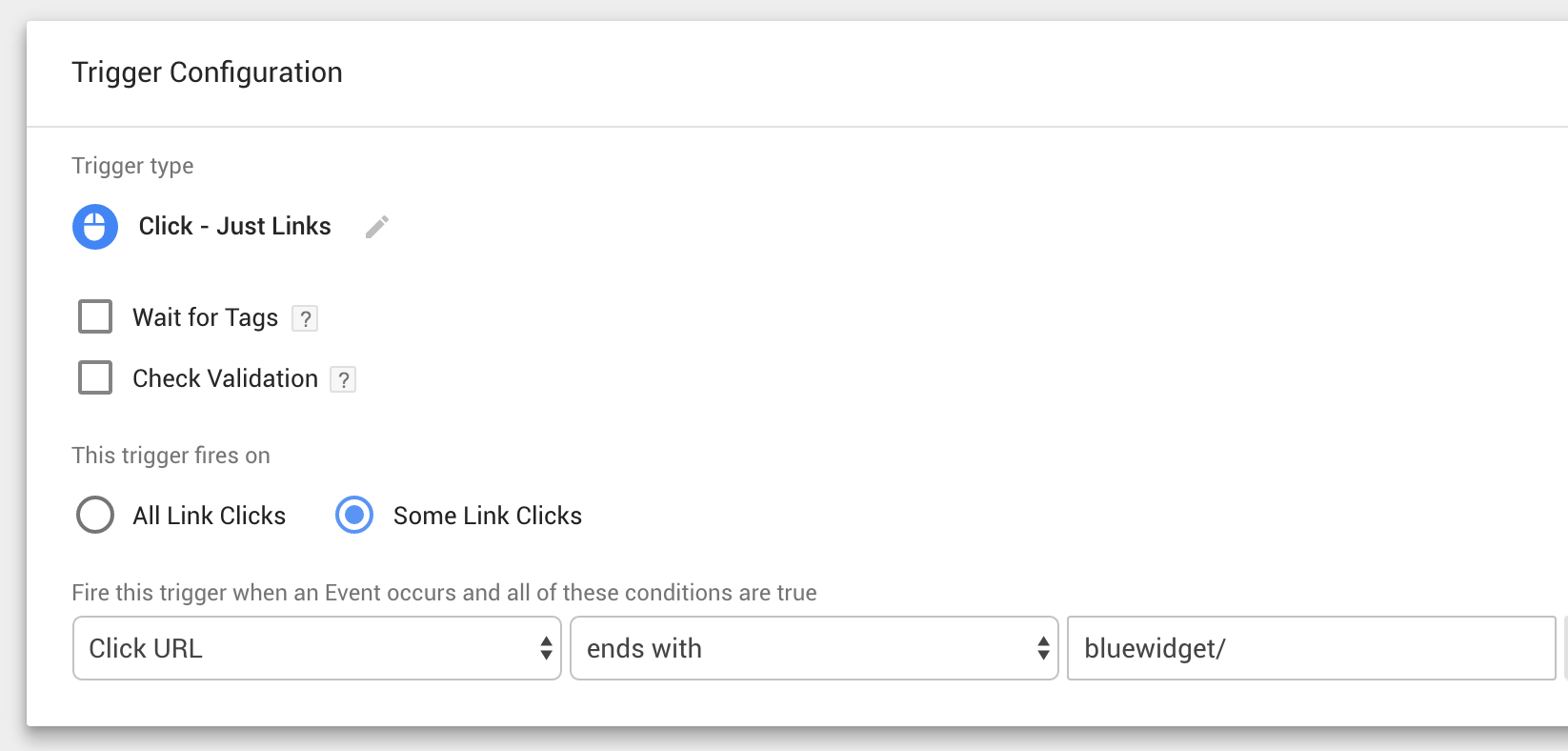The image displays a user interface for configuring triggers. 

At the top, there is a white rectangle with a shadowed border, creating a layered effect with the light gray rectangle behind it. The title "Trigger Configuration" is prominently displayed in bold black lettering. Below this title, a thin, light gray line divider separates the sections. Beneath the divider, the phrase "Trigger Type" is written in smaller light gray font.

A mouse icon featuring a white mouse on a blue background is positioned nearby. Adjacent to the icon, bold black text reads "Click - Just Links." To the right, a light gray pencil icon, pointing downwards to the left, signifies editing options. Below this row, there is an empty checkbox with a gray outline labeled "Wait for Tags," and beside it, a light gray box with a question mark inside.

Further down, another gray empty checkbox is labeled "Check Validation," accompanied by an outlined box with a question mark. In light gray lettering, it says "This trigger fires on:" followed by two tick boxes. The first tick box option, "All Link Clicks," is unselected, while the second option, "Some Link Clicks," is selected, indicated by a blue bullet point inside a blue-outlined box.

The section continues with the instruction, "Fire this trigger when an event occurs and all of these conditions are true," written in light gray text. Below, there are three dropdown menus. The first one reads "Click URL," the second "Ends With," and the third contains the text "blue widget -". The final dropdown menu's text is partially cut off, rendering it unreadable about one-tenth of the way through.